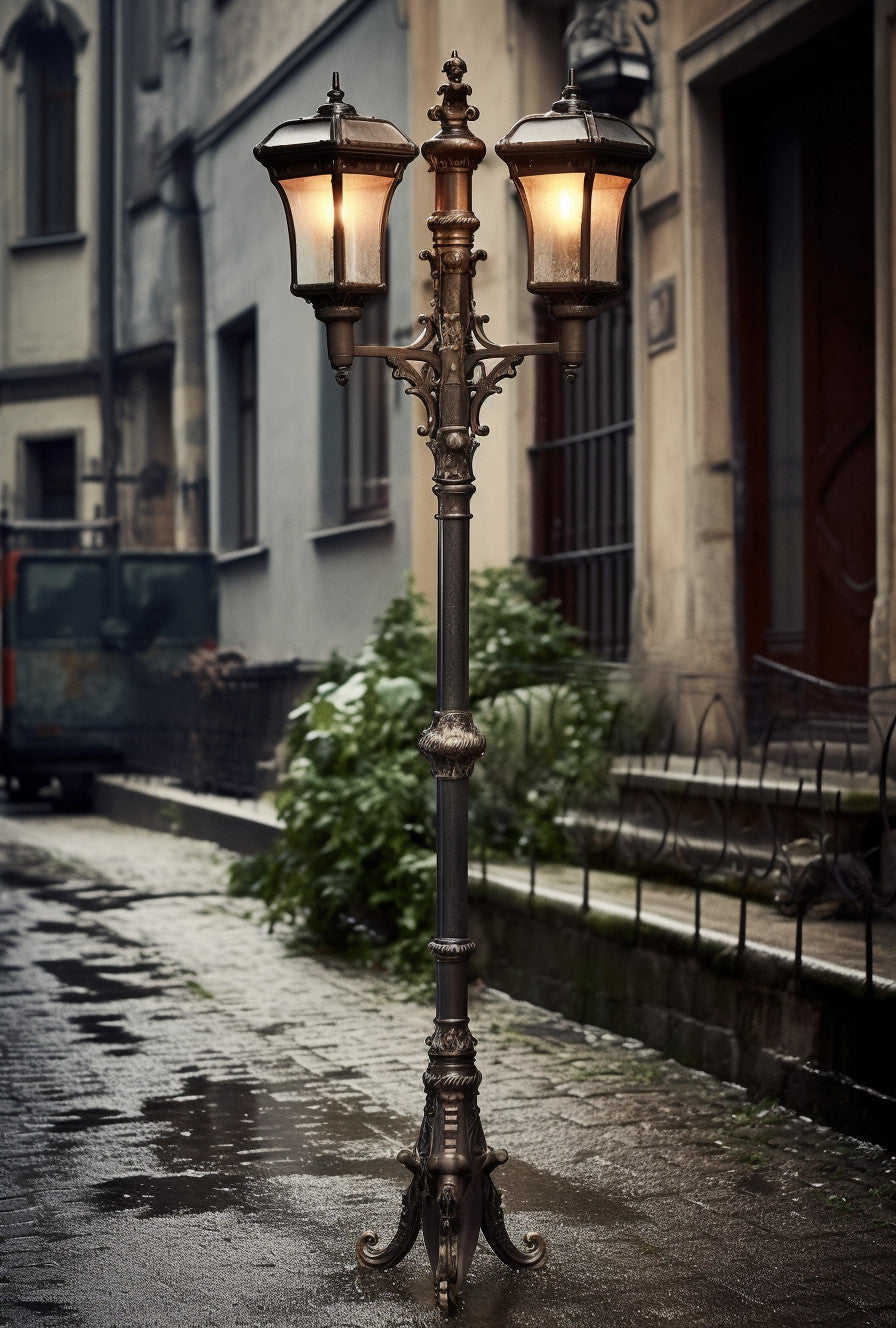The photograph depicts an ornate, classical-style, bronze-colored street lamp positioned centrally on a cobblestone pedestrian walkway. The lamp features a three-legged base that stabilizes it on the wet, puddled pathway, with a singular main pole extending upwards. Towards the top of the lamppost, two elegantly designed arms reach out, each adorned with a glass-enclosed lantern that emits a warm, fire-lit glow. The lamp is intricately decorated from the base to the lanterns, which are topped with small metal roofs. The street is a mosaic of stone bricks still glistening from the recent rain.

In the background on the right side, the image captures a row of townhouses constructed with light brown and gray stones, featuring doorways and a black metal gate. Steps ascend from the street to the buildings, adorned with green plants cascading down towards the cobblestones, adding a touch of nature to the urban scene. The lamppost, with its timeless design, evokes a sense of historical charm amidst the wet, rainy atmosphere.